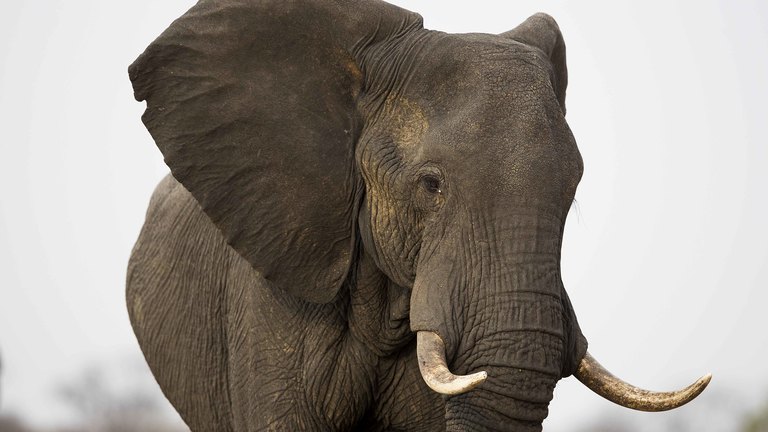The image showcases a vivid close-up of the top half of a gray elephant set against a white background, with notable features taking up most of the center of the frame. The elephant, characterized by its saggy, wrinkled skin and scaly trunk, faces forward. His head is slightly turned to the left, prominently displaying his large, fully open right ear and his expressive right eye, while the left side remains out of sight. Both tusks, curving outward and slightly angled towards the camera, are dirty white in color. The immense size of his ears compared to his relatively smaller body suggests he might be a baby elephant or the photo might have been edited. His coloration is a mix of dark gray and brown, with visible dirt or scarring on his face, adding to the rugged texture of his skin. The image captures an intimate and detailed portrait, with the elephant's attentive posture as if engaged with the viewer.